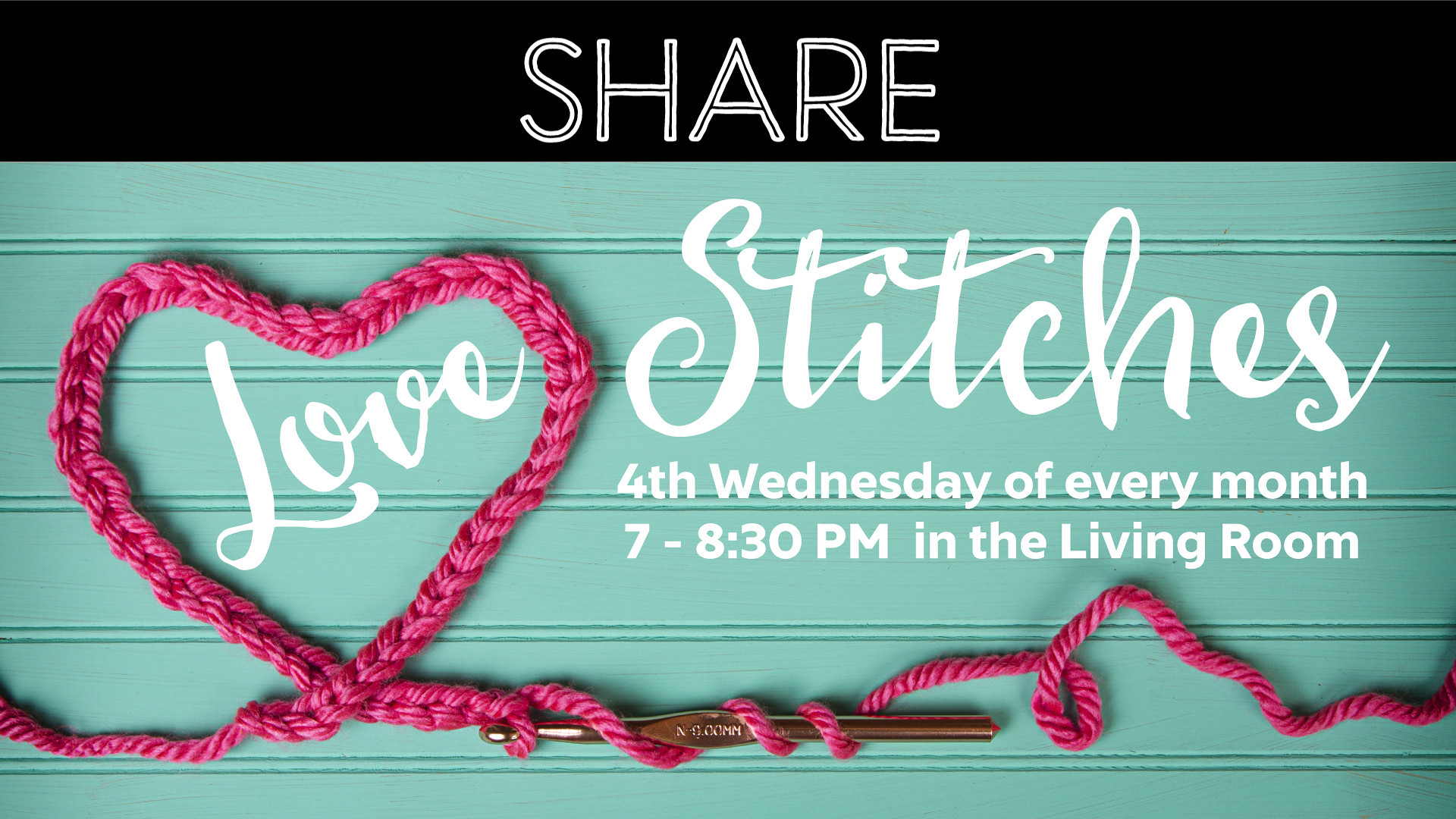The image depicts an advertisement with a beautifully crafted design. It features a heading that reads "Share" in thin-lined, white outline text against a black rectangular background at the top. Below this heading, the centerpiece of the ad is the phrase "Love Stitches," written in a cursive, handwritten-style font in white lettering. The word "Love" is uniquely encircled by a heart made of pink thread or yarn, giving it a sewn-together appearance with a crochet needle visible underneath. This detailing creates a sense of warmth and creativity, akin to a crocheted piece. The background consists of light turquoise or bluish-green wood paneling, adding a rustic charm to the overall design. Beneath the "Love Stitches" text is additional information: "Fourth Wednesday of every month, 7:00 - 8:30 p.m., in the living room," indicating a recurring event. The overall layout is rectangular, emphasizing a blend of creative and communal vibes.